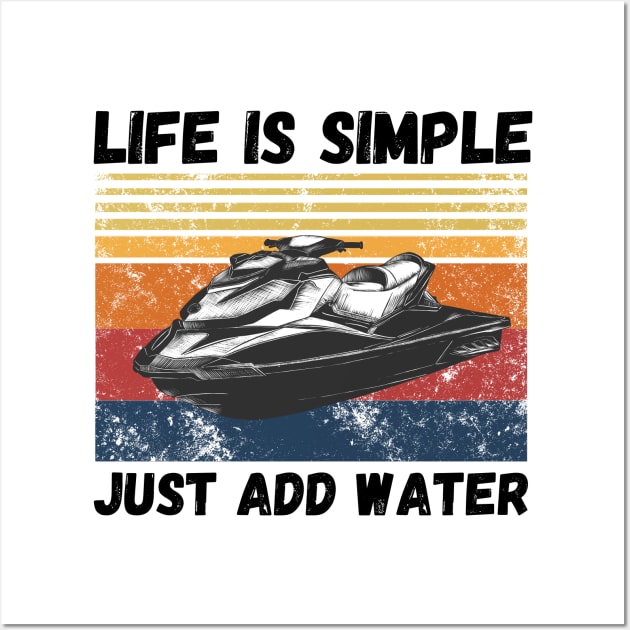The image features a black and white drawing of a sleek jet ski positioned centrally against a background of horizontal stripes. The background exhibits a grungy texture with speckled, crackled lines in varying colors, starting from a dark blue at the bottom, transitioning upward through red, dark orange, lighter orange, and ending with gold at the top. These colored bands become thinner and lighter as they ascend. Bold, black, sans-serif, italicized text at the top reads "Life is Simple," with "Just Add Water" written directly beneath it. A thick white border frames the entire artwork, isolated against a plain white background, emphasizing the central elements. The overall composition reflects a message of simplicity and leisure, encapsulated by the vivid, mottled colors and clean, structured layout.